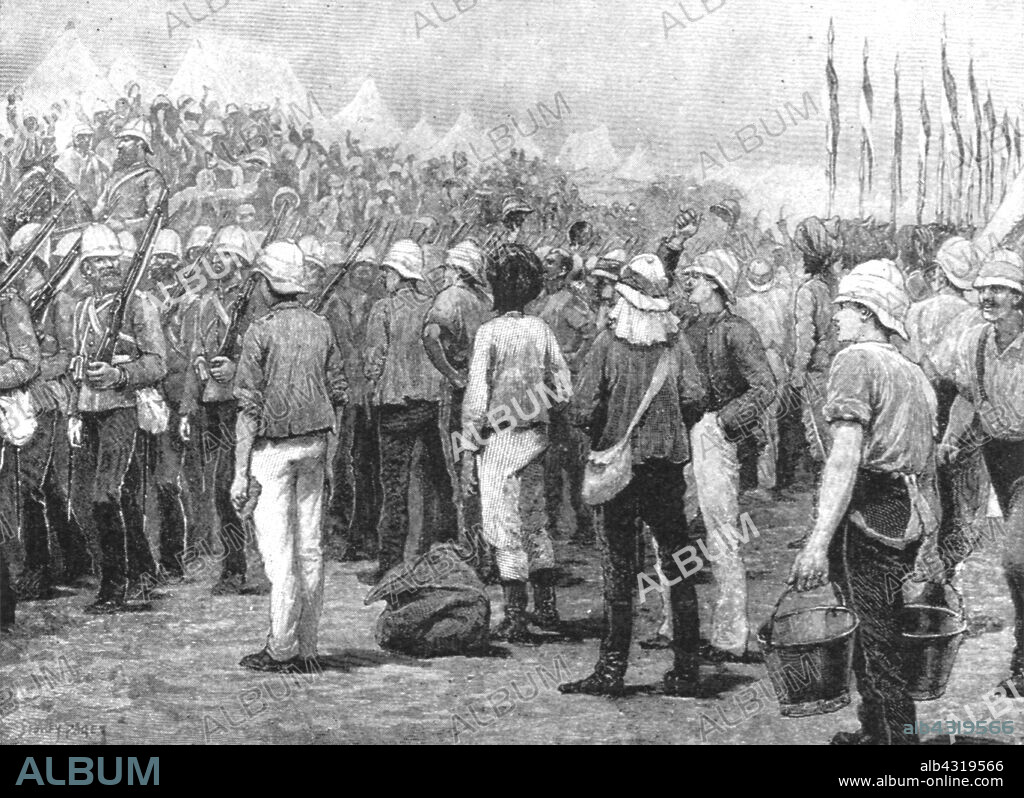This black and white pencil drawing depicts a historical wartime scene featuring a large group of soldiers and civilians. The soldiers, approximately twenty in number, are positioned on the left side, marching to the left. They are dressed in light gray jackets, black pants, and white curved round hats. Each soldier carries a rifle over their left shoulder, supported by their left hand, and wears a strap over both shoulders forming an X. In contrast, the center of the image shows a few civilians, with one man in the forefront carrying two buckets. The background of the scene is filled with blurred images of many people, possibly hundreds, who appear to be both cheering and involved in combat. Flags can be seen wrapped around poles. At the bottom left of the image, blue text reads "ALBUM" and at the bottom right, white text displays "ALB431-9566" along with the website "www.album-online.com." The word "album" is also catty-cornered across the picture multiple times.